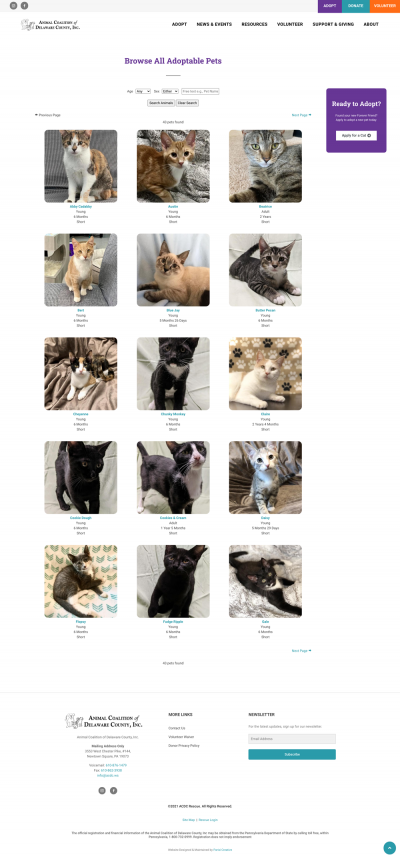This screenshot features a user interface with a clean white background and a light gray rectangle spanning the width of the screen at the top. On the left side of this gray header, there are two gray circular icons, while on the right, three colored rectangles are neatly aligned: a purple rectangle, a blue-green rectangle, and an orange rectangle. Beneath this header is a line of very small text, which is followed by a purple, centered statement reading "Browse all adoptable pets."

Below this statement, two lines in gray text provide additional context or instructions. The main section of the screen displays a grid of pet images, arranged in three columns and five rows, predominantly featuring cats.

Adjacent to the top-right corner of the pet images grid is a purple box containing a white rectangular button. Below the pet images grid, a white rectangle houses a logo and some text in the left-hand corner. This section is divided into two columns with bold black labels, and on the right side, there is a blue-green button. The overall layout is organized and visually structured, providing a clear path for users to explore adoptable pets.